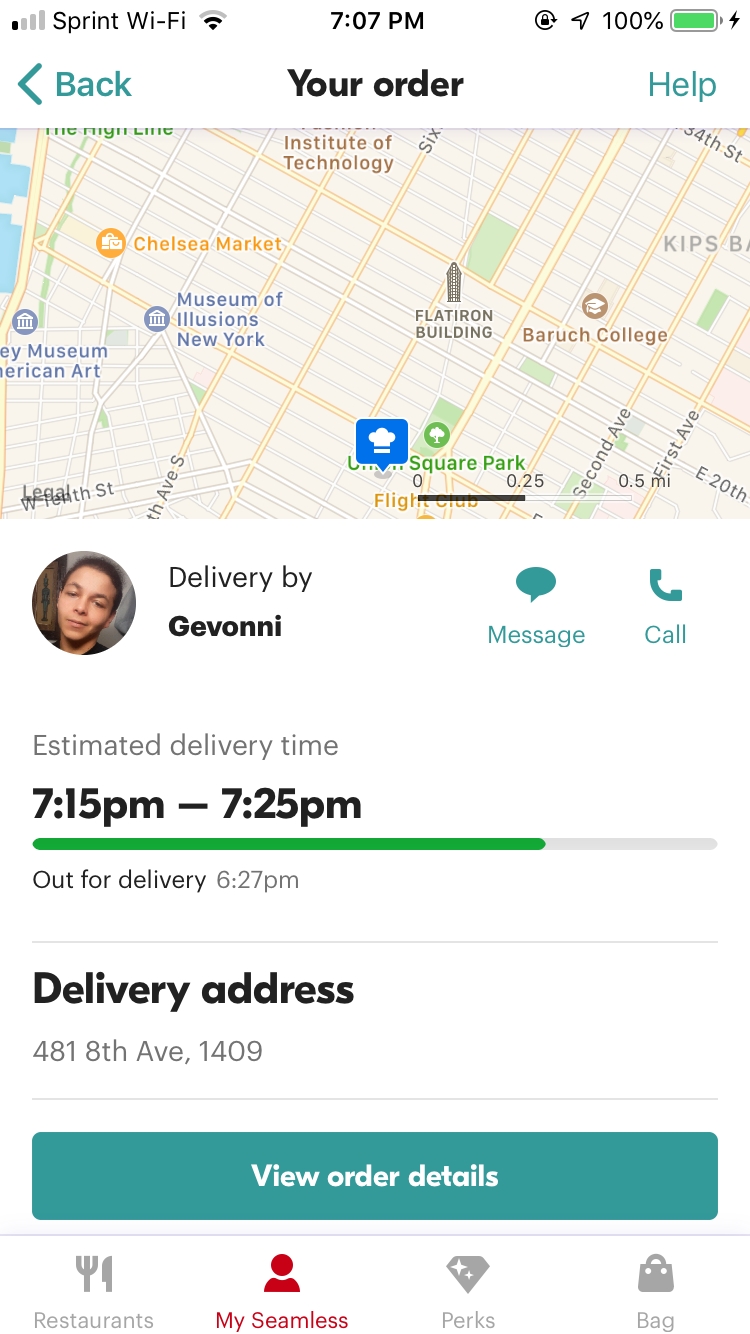This screenshot captures the detailed interface of a smartphone app, likely related to food delivery. Situated in the upper left-hand corner, iconography indicates cellular signal strength, followed by the "Sprint Wi-Fi" label. Adjacent to this, a Wi-Fi strength icon is visible. Centrally positioned is the time display, showing "7:07 PM", flanked by a location services icon on the right, and a fully green battery icon indicating a 100% charge.

Beneath the time display, "Order" is indicated prominently in the center. On the left side is a "back" option denoted by a less-than sign (<), enabling return to the previous screen. On the far right, the word "help" appears in greenish letters. Below this section is a map, akin to a Google map interface. Further down, there's a small circular photo of a male, along with text that reads, "Delivery by Giovanni." To his right are options for messaging or calling.

In a gray font just below this, the estimated delivery time is listed as "7:15 PM - 7:25 PM" in black. The progress bar immediately underneath is about three-quarters full with a green line. To the right of this bar, "Out for delivery" is shown with the timestamp "6:27 PM."

Following that, the "Delivery address" is shown in black font, with "481 8th Ave, 1409" in gray font below. A button labeled "View order details" in white font appears beneath this section. At the bottom of the screen, there are four menu options: "Restaurants," "My Seamless" (highlighted in red), "Perks," and "Bag".